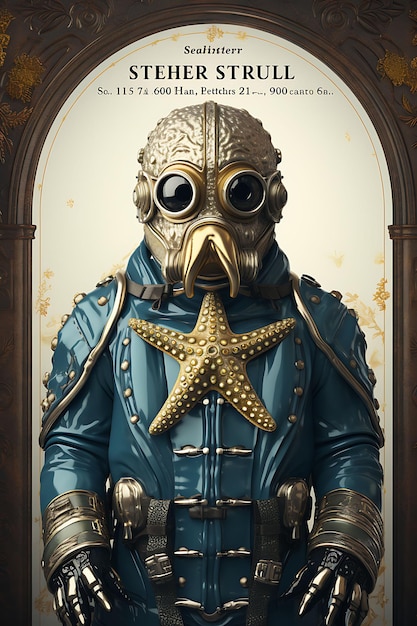The image depicts a fantastical, science fiction-steampunk themed creature named Steher Strahl, as indicated by the text at the top in a foreign language. This awe-inspiring character is adorned in a blue, armored suit featuring a distinctive starfish emblem across the chest. The suit is detailed with insignia reminiscent of military or superhero armor. The creature is helmeted, with bug-like goggle eyes and a metal brain casing, hinting at either a futuristic augmentation or an individual wearing an elaborate costume. Clad in gloves that resemble metallic bones or claws, the character exudes an otherworldly and intimidating presence. The background is primarily white, accented by small yellow, floral-like patterns, and framed by a black or very dark brown doorway, creating a stark contrast that highlights the striking appearance of Steher Strahl. Adding to the mysterious allure, there are numbers and text—potentially an address or additional information—formatted atop the image, contributing to the enigmatic and intriguing nature of this visual presentation.